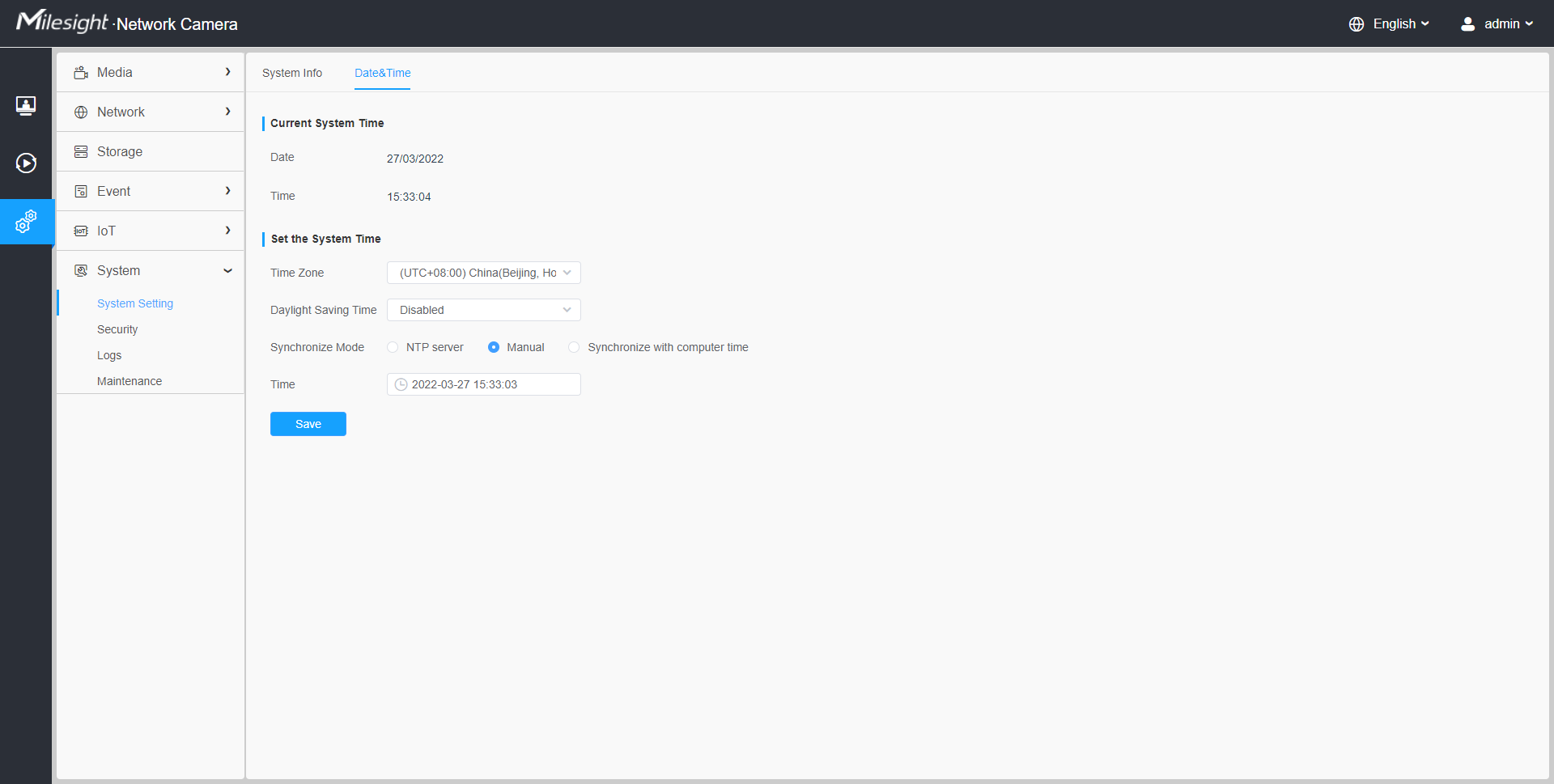A screenshot of a computer screen displaying the interface of a Mile Site Network Camera. The interface is framed by a black vertical sidebar on the left and a black horizontal bar across the top. In the upper left corner of the screen, the text "Mile Site Network Camera" is prominently displayed in white. On the upper right, there's a dropdown labeled "English" with an icon to its left, and adjacent to this, a user icon followed by the text "admin" with an arrow pointing down.

The vertical black sidebar on the left contains three icons, with the third icon highlighted in blue, indicating the current selection. Adjacent to this sidebar, the main area of the screen features a white vertical menu, listing options such as "Mode," "Network," "Storage," "Email," and "Systems," with corresponding arrows to the right of each item. A vertical light gray line divides this menu from the other content on the screen.

The interface to the right of this menu is divided into three sections. The top section appears to be a header area. Below this, two sections are delineated by bold black titles, each accompanied by their own content: the first section includes two lines of text, while the second section includes four lines of text. Both sections feature search bars to their right, providing options for quick access or filtering within these categories.